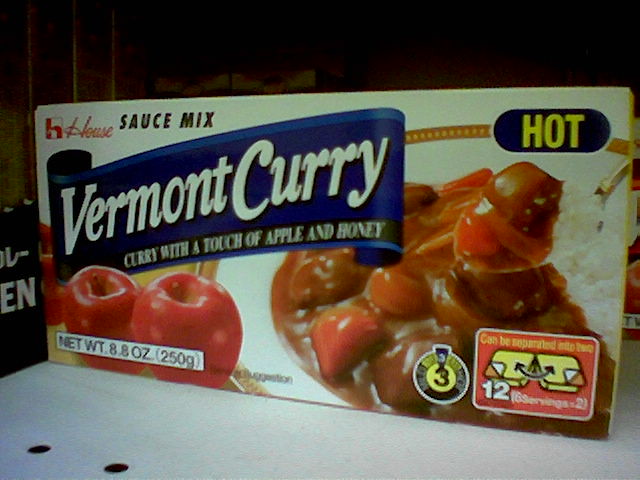The photograph depicts a product package set against a black background, which extends across the entire image. The central focus is a box of House Sauce Mix labeled "Vermont Curry." Prominently displayed on the box, there is a dark blue banner with the words "Vermont Curry" in bold white letters. Beneath this, it reads "Curry with a touch of apple and honey" in smaller white capitals. The top left corner features the brand name "House" in red script, accompanied by a small lowercase "h." To the upper right, the word "hot" appears in yellow capital letters within a dark blue oval. Directly below, there's an image likely illustrating the sauce served over white rice alongside vegetables, suggesting a serving idea. Adjacent to this, the packaging indicates it yields 12 servings and includes a small icon resembling a timer, stating a microwave time of 3 minutes. At the bottom left, the box shows two red apples, hinting at the apple and honey flavor, with the net weight specified as 8.8 ounces (250 grams).